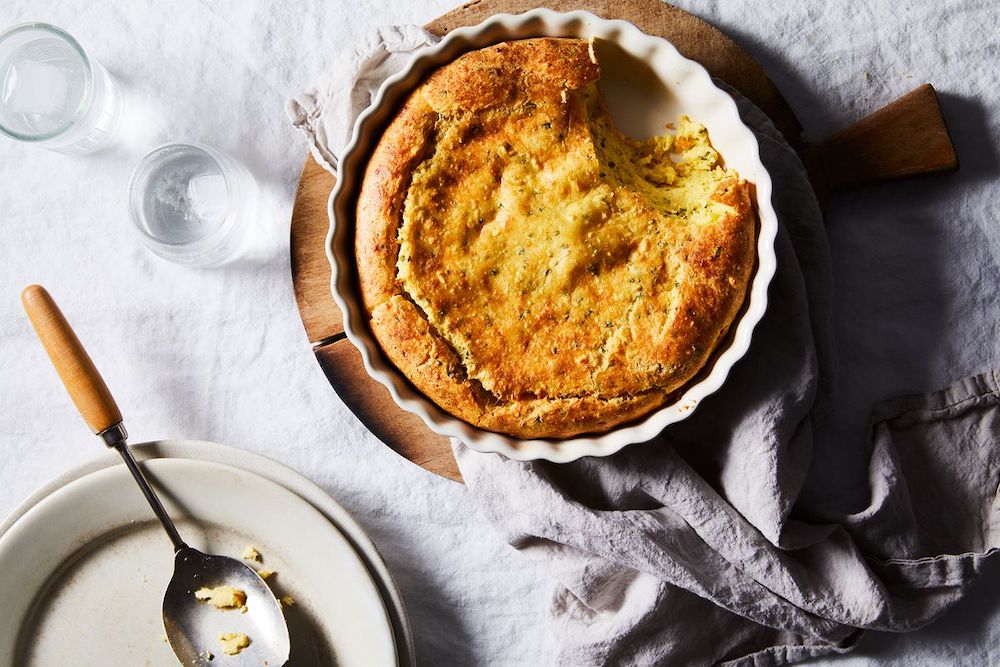In this detailed color photograph, we have a visually appealing top-down view of a kitchen setting, featuring several distinct objects laid out on a white linen tablecloth. At the center of the image is a golden-crusted baked item, possibly cornbread or a souffle, housed in a white baking dish with a ruffled edge. This dish is set on a round wooden cutting board, and a significant scoop has been removed from the top right, revealing the soft interior.

In the bottom left corner, there are two nested white bowls. The inner bowl contains a few crumbs and a stainless steel serving spoon with a wooden handle, positioned toward the middle left of the image. Above these bowls, and still in the upper left quadrant, are two clear, translucent water glasses.

The scene also includes a white cloth napkin in the bottom right corner, adding to the sense of a recently enjoyed meal. The overall color palette features shades of white, clear, brown, yellow, and orange, contributing to the warm and homey atmosphere of what appears to be a kitchen table setting. This photograph exemplifies food photography clarity and realism, capturing a moment that invites curiosity and appreciation.